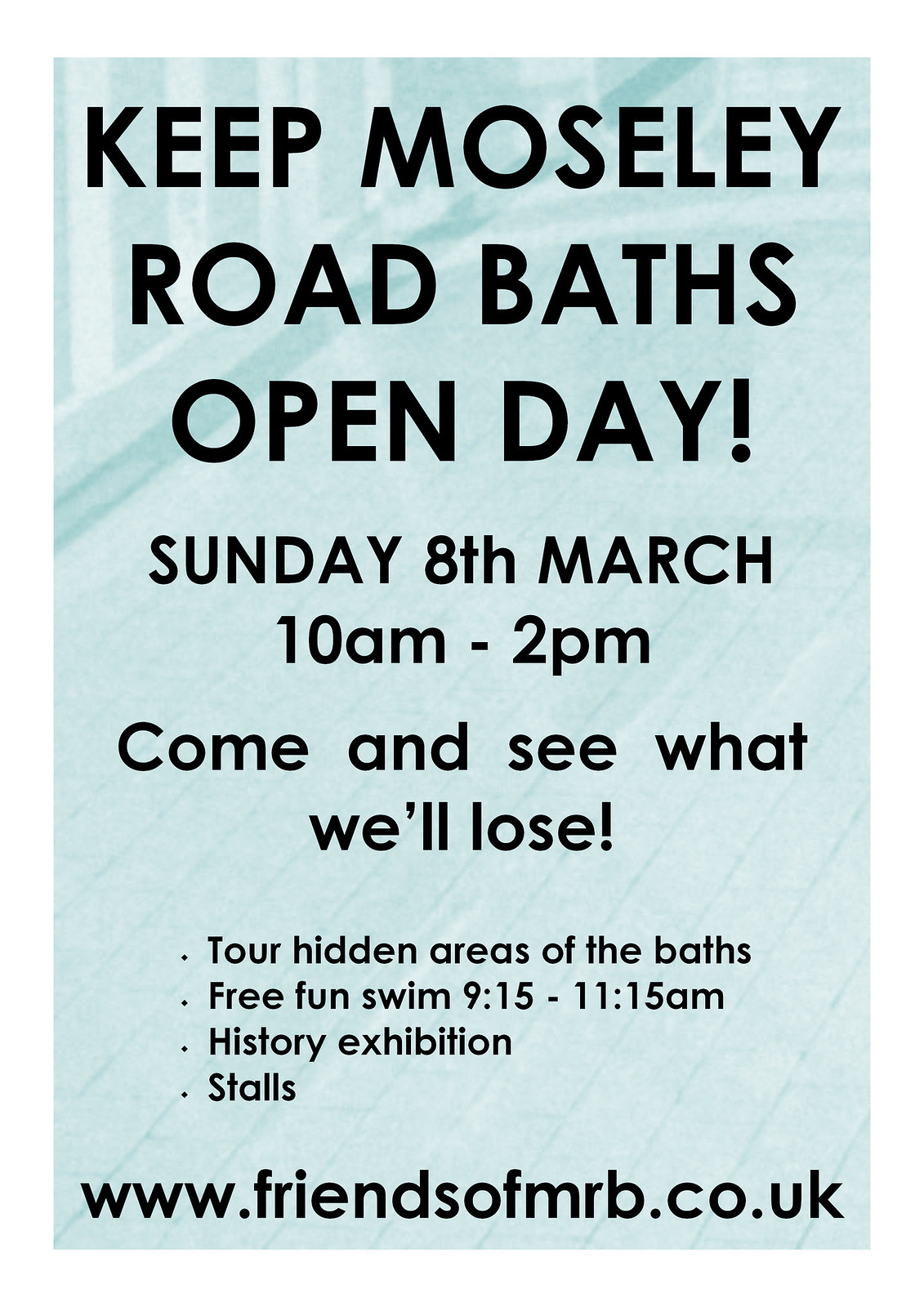The advertisement features a soft, light blue or light bluish-green background that mimics the appearance of wood or a deck, accented by a railing at the top, giving it the feel of a boardwalk. Bold black text at the top announces, "Keep Moseley Road Baths Open Day!" and below it, in slightly smaller black font, the event details are given: "Sunday, 8th March, 10am to 2pm." The next line reads, "Come and see what we'll lose!" which is followed by a bullet-point list detailing the activities: "Tour Hidden Areas of the Baths," "Free Fun Swim, 9.15am to 11.15am," "History Exhibition," and "Stalls." At the bottom of the advertisement, a website address is provided: "www.friendsofmrb.co.uk." The overall layout focuses solely on this detailed announcement, ensuring clear communication of the event's purpose and schedule.